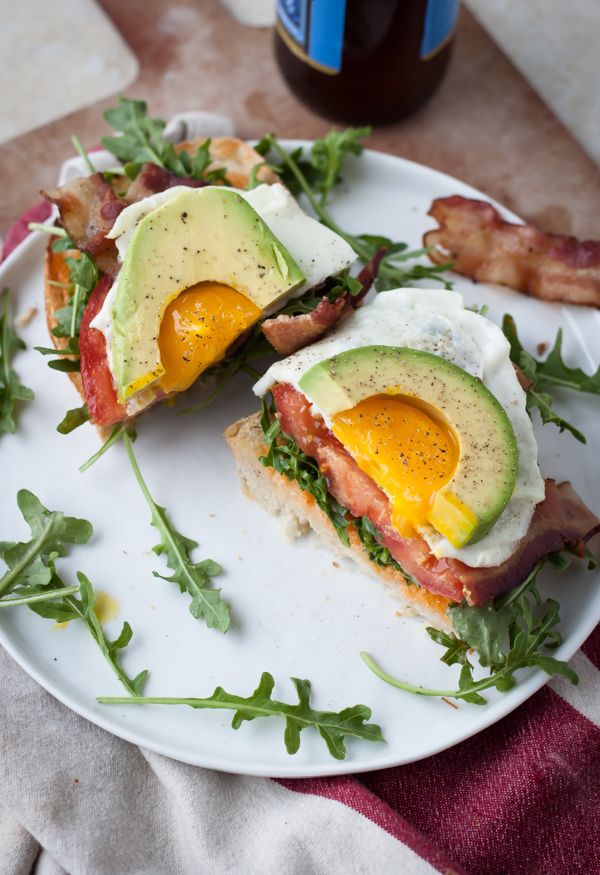In this image, we see a detailed close-up view of a breakfast sandwich artfully arranged on a white circular plate, which is set on a red and white striped cloth atop a brown table. The sandwich, made from toasted white bread, is cut in two, with one half positioned at the top of the plate and the other half to the right. The sandwich is layered with fresh arugula, a thick slice of tomato, crispy bacon, and a sunny-side-up fried egg adorned with a curved slice of avocado crowning the yolk, likely seasoned with salt and pepper. The plate is garnished with additional scattered arugula leaves and a piece of bacon positioned on the upper right. Just above the plate, a brown bottle with a blue label is partially visible, adding to the composition. The combination of colors and textures creates an appetizing and visually appealing presentation.